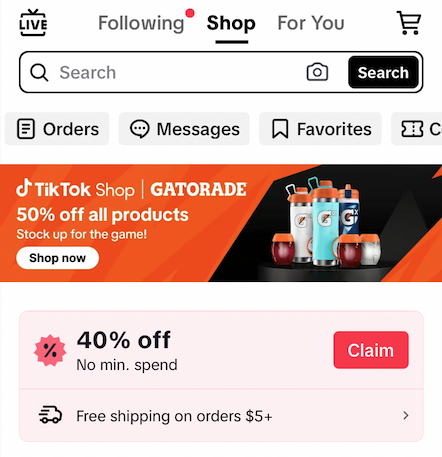The image is a screenshot from an online shopping interface, likely from TikTok Shop. The screenshot includes multiple UI elements, starting in the upper left corner where a "Live" icon is displayed instead of a traditional TV icon with antennas. It indicates "Following" with a red dot next to it. Immediately below, there are options labeled "Shop," which is underlined and in bold, and "For You" next to a shopping cart icon. 

Beneath those tabs, there is an empty search bar followed by navigation options for "Orders," "Messages," and "Favorites." 

Further down, an orange advertisement banner reads "TikTok Shop: Gatorade 50% Off All Products." The banner encourages users to "Stock up for the game and shop now," featuring an array of Gatorade containers. It also mentions "40% off no minimum spend" and includes a red button to claim this offer, highlighting "Free shipping on orders of $5 or more."

Overall, the advertisement campaign is designed to entice viewers, likely watching a live TV show online, to purchase beverages in preparation for an upcoming game, leveraging significant discounts and free shipping as incentives.